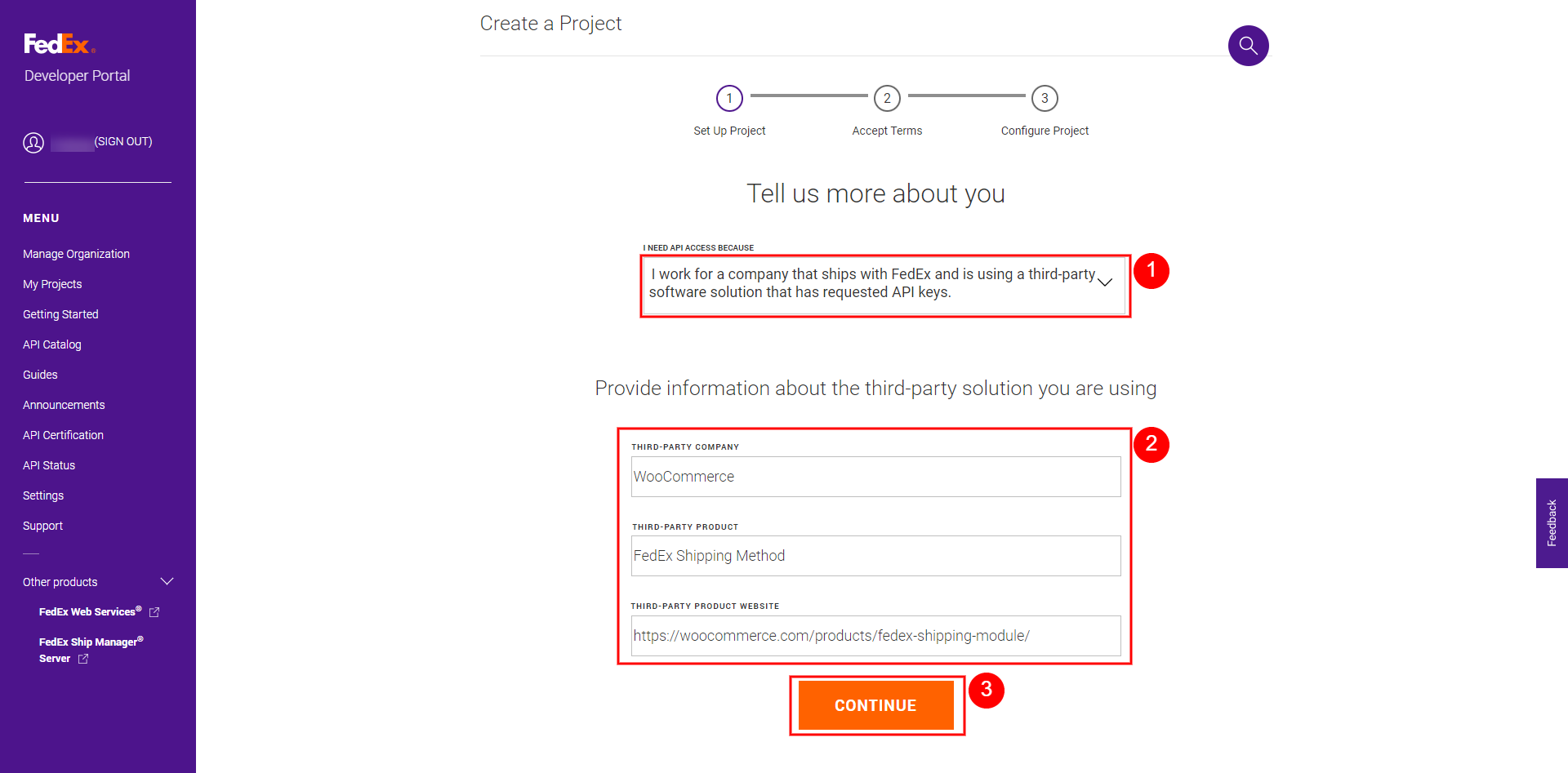The image depicts a page from the FedEx Registered Developer Portal. On the left side of the interface, a vertical menu is visible, featuring various icons and buttons. The menu items listed include:

- Manage Organization
- My Projects
- Getting Started
- API Catalog
- Guides
- Announcements
- API Certification
- API Status
- Settings
- Support
- Other Products
- FedEx Web Services
- FedEx Ship Manager

The user's name is obscured, either blurred out or streaked over for privacy. In the main section of the page, there are instructions for creating a project, divided into three steps:

1. Set up Project
2. Accept Terms
3. Configure Project

The form instructs the user to provide information about their usage, specifically asking them to describe their company’s relationship with FedEx and mention any third-party software solutions they are utilizing that require API keys. 

The color scheme of the page includes orange, black, white, and purple, which are consistent with the FedEx branding.